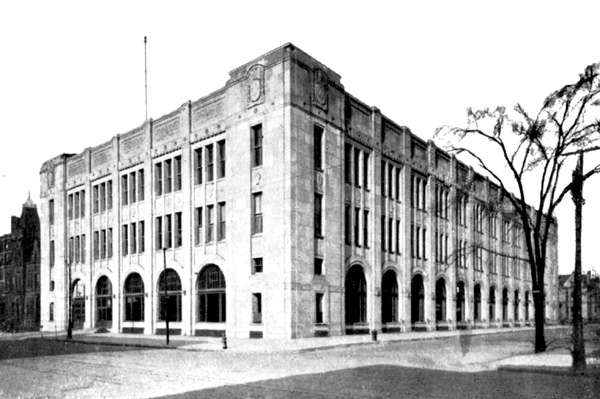This black-and-white photograph features a striking early 20th-century building, possibly from the 1910s to the 1930s, located on the corner of a large urban plaza. The building, constructed in a sturdy, likely brick material, showcases art deco architectural style with intricate decorative trim adorning the top layer. It spans three stories with narrow, vertical windows spreading across its facade, similar to federal or neoclassical designs. The lower floor is distinguished by arched glass windows that wrap around the base, suggestive of commercial spaces. From the perspective of the image, a lamppost and a mostly bare-branched tree are visible on the right-hand side, accentuating the corner view. The scene lacks any human presence, highlighting only the detailed architecture and sparse vegetation around the structure. Edges of other buildings are faintly visible in the background, suggesting a dense urban setting, possibly indicating the building's role as a bank, government office, or library. A cement walkway encircles the building, bordered by patches of grass.